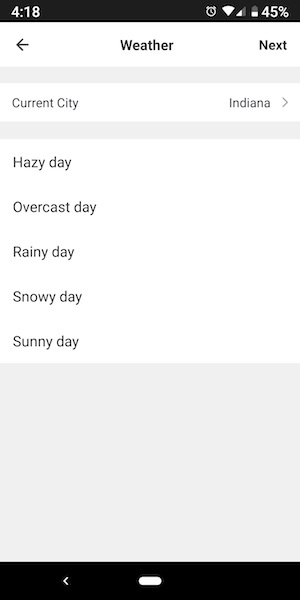This mobile screenshot was taken at 4:18, depicting an alarm that is currently set. The simplified icons at the top of the screen—comprising an alarm icon, a WiFi icon with full signal, mobile data bars showing partial connectivity, and a battery at 45%—suggest the phone is an Android device with customized, less detailed icons.

The screenshot showcases a weather app interface. At the top of the app, there are navigational controls: a back button, a label indicating "Weather," a "Next" button, and a field labeled "Current City," which is editable but currently displays "Indiana" alongside an arrow for selection.

The main section of the weather app lists various weather conditions: "Hazy day," "Overcast day," "Rainy day," "Snowy day," and "Sunny day." It is unclear if these options are for manual weather entry or selection.

At the very bottom of the screen are the standard Android navigation buttons: the menu (or home) button and a back arrow. The overall design of the interface is simple and user-friendly, favoring ease of selection and minimalistic visuals.